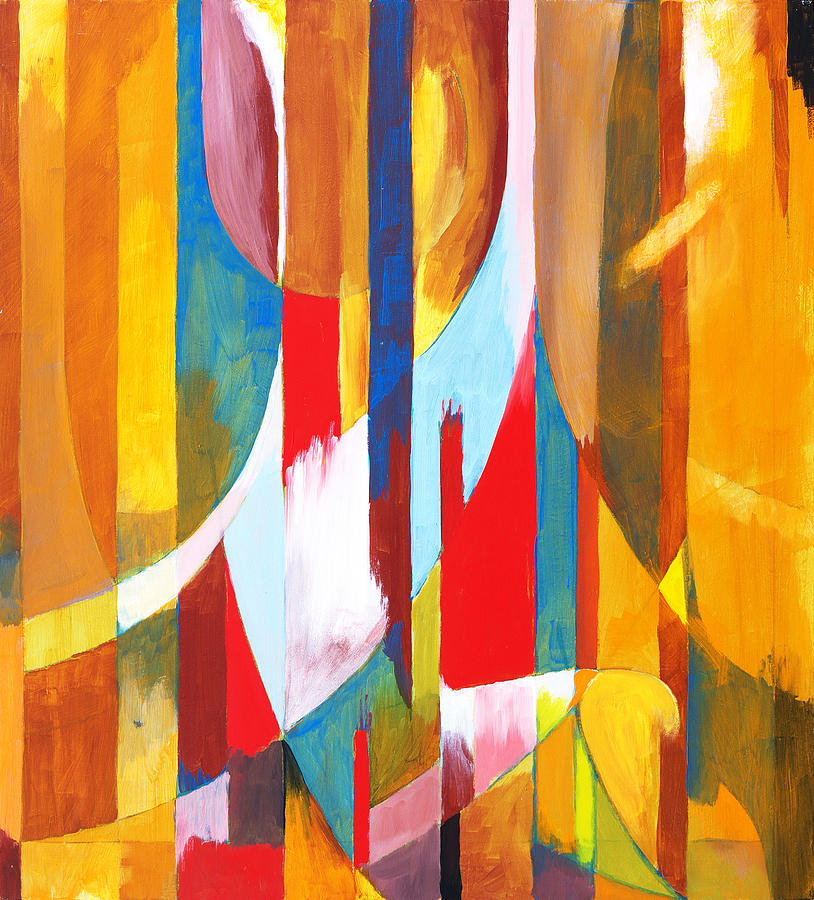This vertically oriented abstract painting features a dynamic array of bold colors and forms, dominated by a series of vertical bars that span the entire height of the canvas. Prominent colors include vibrant shades of orange, yellow, blue (ranging from royal to navy to light blue), red, green, and brown. The central composition is disrupted by swirling patterns interspersed amongst the vertical lines, creating a complex visual texture. A striking dark blue bar descends through the middle, intersected by red and lighter blues. Towards the right, various brown and yellow hues emerge, while the left side is noted for white outlines delineating the interplay between colors. Despite the chaos of curves and swirls winding through the painting, the primary impression remains one of vertical continuity. Interestingly, the absence of an artist’s signature leaves the creator of this intricate work anonymous.